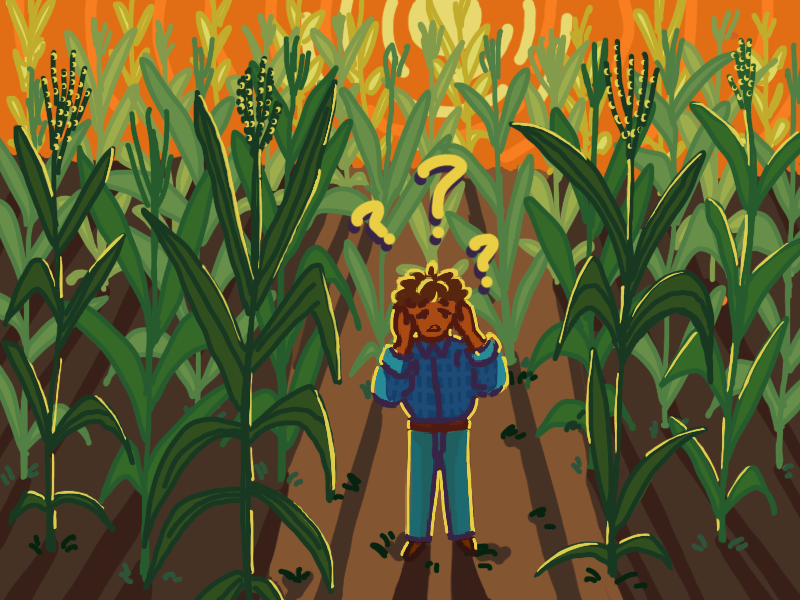This digital artwork depicts a child standing in the middle of a cornfield, surrounded by tall blue-green cornstalks that frame the scene on both sides and behind them. The child, positioned towards the bottom center of the image, stands on brown dirt, which has lighter and darker patches. They are dressed in a blue outfit that includes a blue plaid shirt, blue jeans, a plain brown belt, and brown pointy shoes. The child has a simply designed face with an orange hue, brown hair tinged with yellow, and a worried expression, their orange hands raised to their head. Above their head are three floating yellow question marks with shadows, indicating confusion or uncertainty. In the background, an orange sky transitions to a picturesque sunset with a yellow sun. The artwork, done in a simplistic and cute cartoon style, evokes a sense of being lost or disoriented in a corn maze.